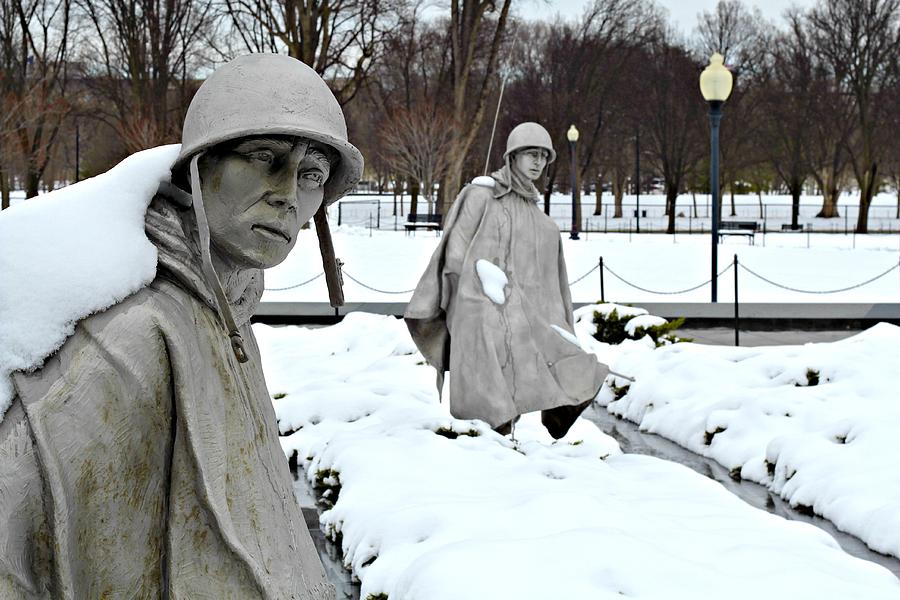This photograph captures a poignant winter scene at what appears to be the Vietnam Memorial in Washington. It features two gray, lifelike statues of soldiers wearing bucket helmets with chin straps and thick, draped ponchos or capes—fashioned to represent the harsh conditions they endured. The soldiers are portrayed leaning backwards and gazing into the distance, with meticulously sculpted faces that exhibit a profound expression in their eyes. The closer statue in the foreground appears almost within arm's reach, while the second statue stands a few feet behind and to the right.

The statues are set in a snow-covered park, where the ground is fully blanketed in white. The background reveals several leafless, brown trees, a black streetlight topped with a yellow bulb, fencing, and benches that are scattered around. Snow adorns parts of the statues, particularly sticking to the soldiers' backs and elbows, while some snow is melting on the sidewalk around them, enhancing the sense of cold.